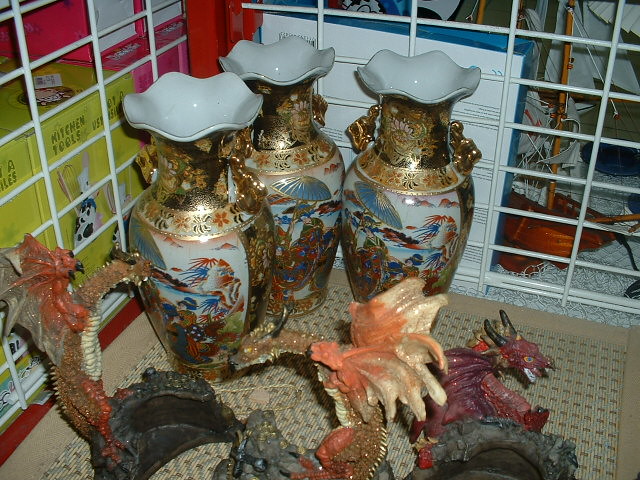This detailed photograph captures a display of three ornate Asian-style ceramic vases artfully arranged in a white metal cage, resembling a storage or clearance area. The vases are prominently decorated with intricate gold floral designs and oriental patterns, and each vase features ornate gold handles and fluted, scalloped rims. The vases, which taper towards their tops, sit on a brown and light tan-colored mat with perforations. In front of the vases, there are three dragon sculptures, each distinct in color: one in dark red, another in golden hues with orange wings, and the third in a deeper gold-orange shade. A closer inspection of the background reveals various boxes and other items stored within the cage, suggesting a retail or storage setting.